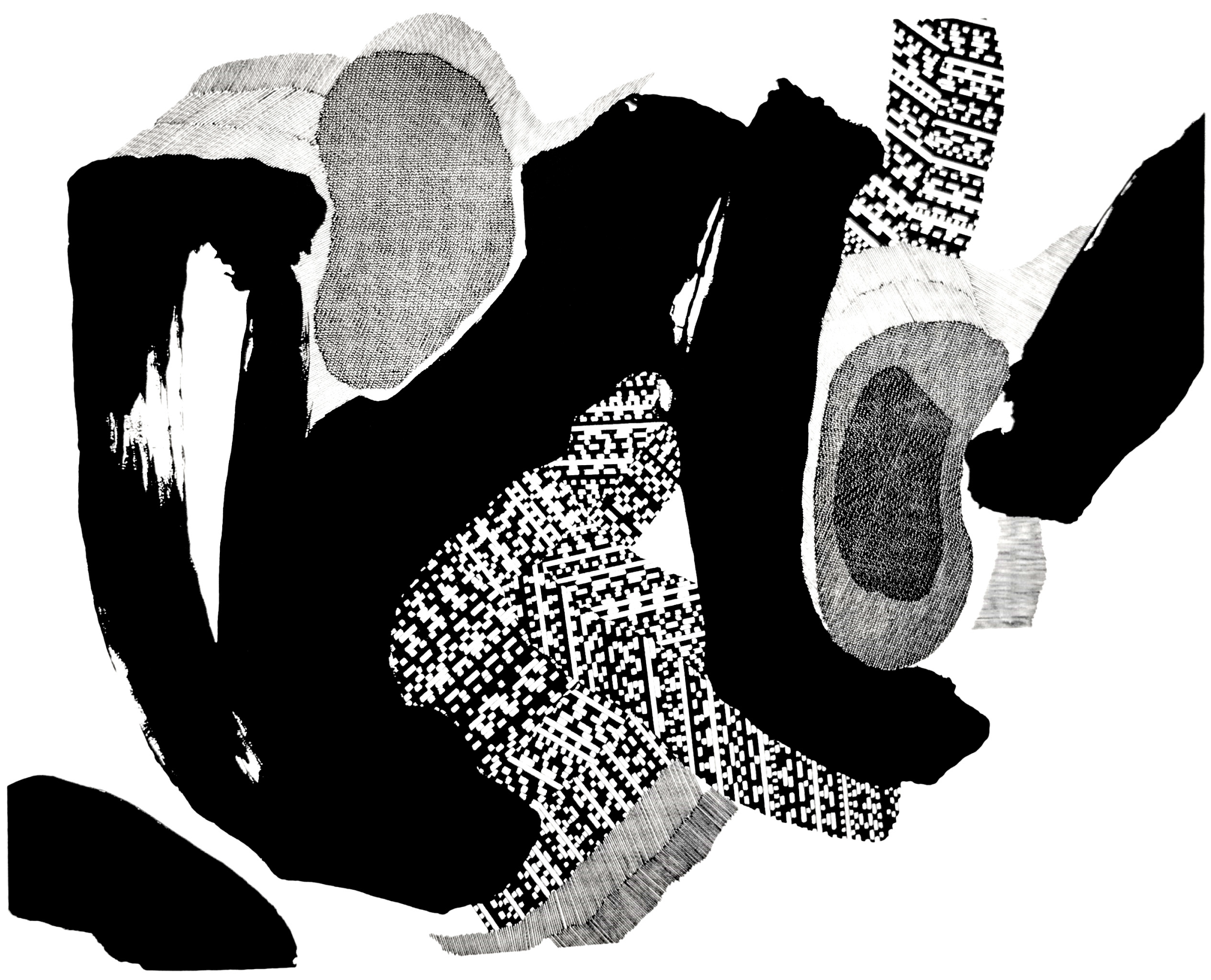The image showcases an abstract artwork composed entirely of black and white elements on a white background. Dominating the composition are two circular blobs and sweeping, wide brushstrokes of solid black. Amidst these bold strokes, an intricate repeating pattern emerges, resembling cloth but remaining an abstract design. Along the left bottom corner, there's a black shape that resembles a shoe or slipper, with noticeable black and white checkered and fringed details. Towards the middle, a dark line runs vertically, accompanied by a QR code-like pattern and additional black and white stripes at the bottom. At the top, fuzzy images and darker patches accented by lighter borders blend into the mix, while another thick black line, evocative of a marker stroke, extends from the right side, contributing to the chaotic yet compelling visual tapestry.